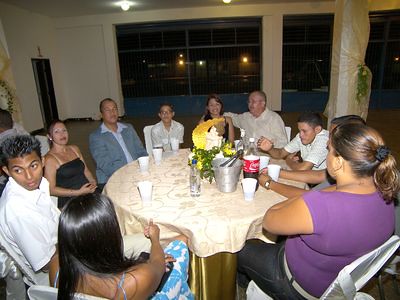The image depicts a lively gathering taking place in a brightly lit celebration hall. A group of 10 to 12 people, dressed in a mix of casual and formal attire, are seated around a circular table adorned with a dual-layered tablecloth: the top layer is a light beige or cream color, with an elegant golden tablecloth beneath it. The table is decorated with a central floral arrangement featuring green leaves and yellow flowers, enhancing the festive atmosphere. Scattered around the table are numerous white plastic cups, a two-liter bottle of Coca-Cola with its distinct red label, an ice bucket likely containing drinks, and a small metal bucket. The surrounding setting includes white chairs, large glass windows allowing natural light to illuminate the scene, white pillars, an overhead lighting system, and glimpses of streetlights or lights from nearby buildings visible through the windows. The overall scene suggests a party or get-together, with a spacious dance floor or open area evident in the background, setting the stage for a joyous and celebratory occasion.